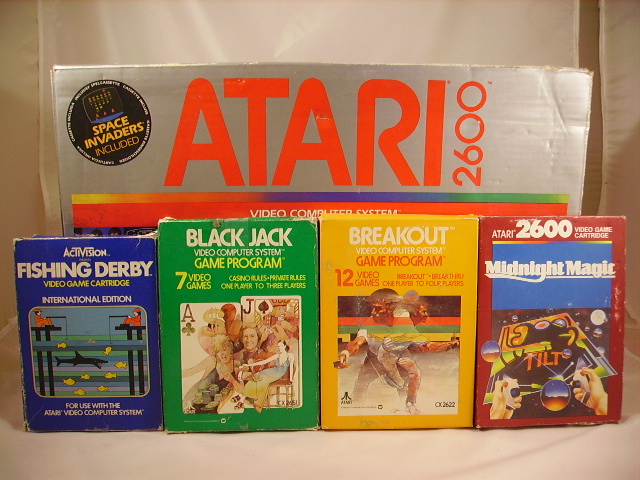This is a vibrant, color photograph showcasing a vintage Atari 2600 gaming system in its original packaging. Prominently displayed on the box is the iconic Atari logo and branding, clearly indicating it is the 2600 model. Attached to the front of the package is a small sticker highlighting that the classic game "Space Invaders" is included with this system. In front of the box, a variety of used Atari game cartridges are neatly arranged and presented as if for sale. These games include "Fishing Derby," "Blackjack," "Breakout," and "Midnight Magic," each in their respective individual packaging. The entire setup resembles a comprehensive eBay listing, meticulously organized to entice collectors and retro gaming enthusiasts looking to purchase this nostalgic bundle.